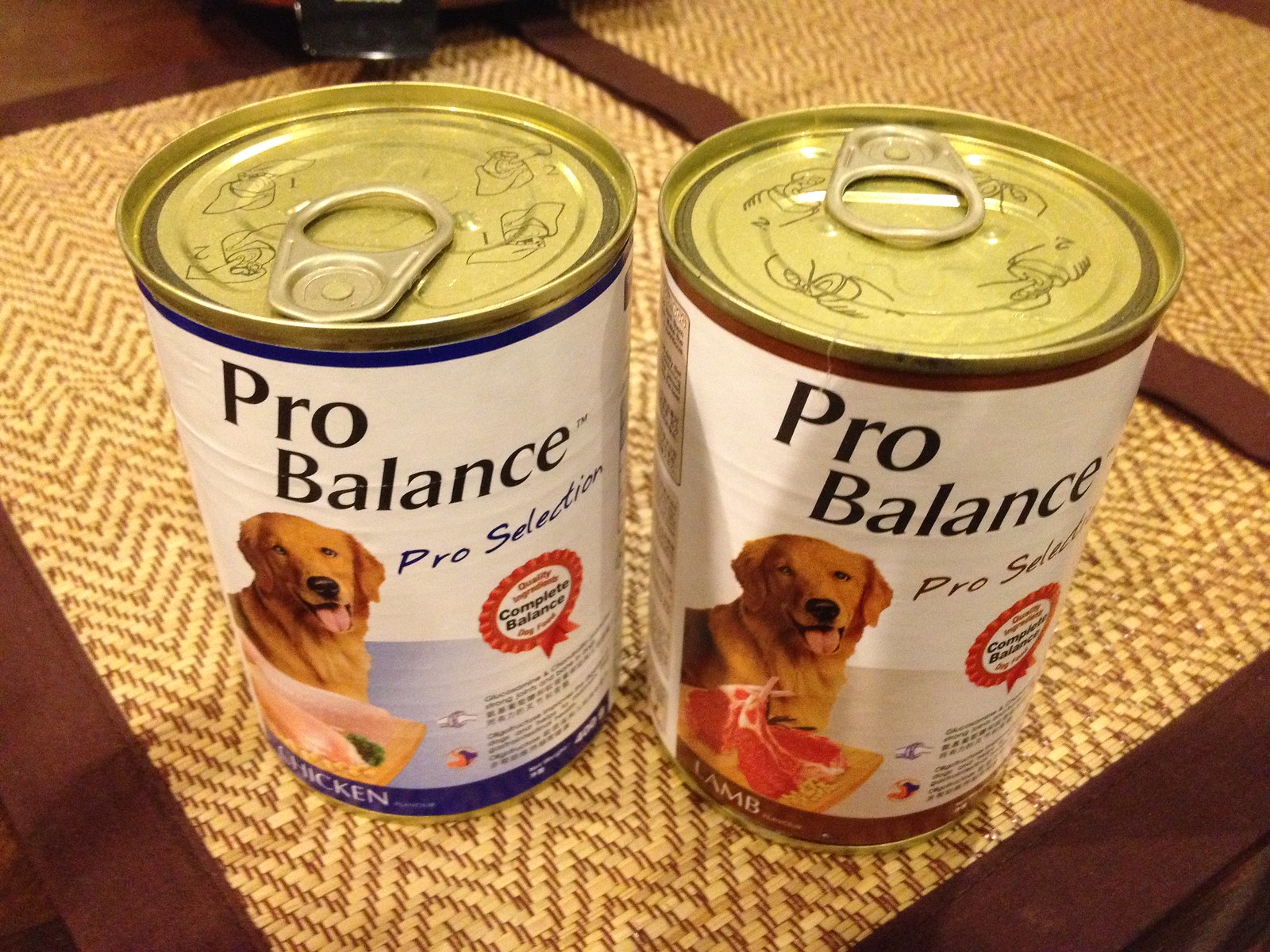This detailed photograph showcases two cans of Pro Balance dog food, prominently placed on a placemat atop a wooden table. The two cans feature different flavors yet belong to the same brand. The can on the left, adorned with blue accents, contains a chicken-flavored dog food and displays an image of a golden retriever alongside a chicken breast. In contrast, the can on the right, which features brown accents, offers lamb-flavored dog food and portrays the same golden retriever next to a rack of lamb. Both cans are labeled "Complete Balanced" and are equipped with pop-top lids, making them easy to open without a can opener.